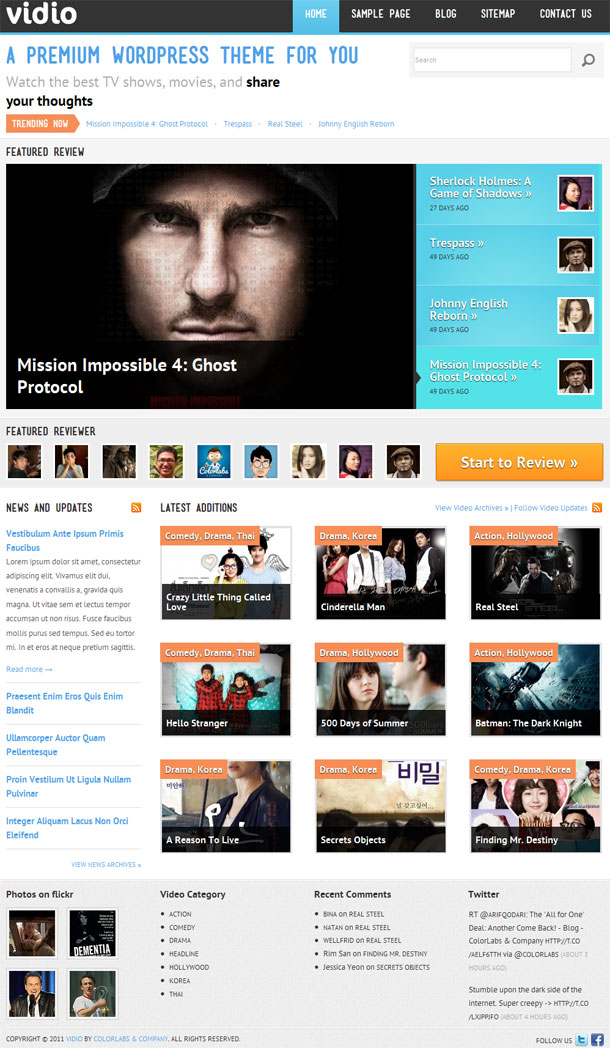The upper left corner of the webpage displays the text "VIDIO". To the right, navigation options include "Home", "Sample Page", "Blog", "Sitemap", and "Contact Us" with "Home" highlighted in blue. Below this, a tagline reads, "A premium WordPress theme for you. Watch the best TV shows, movies, and share your thoughts." 

Beneath the tagline, a section titled "Featured Review" showcases an intense close-up of Tom Cruise, promoting the movie "Mission Impossible 4: Ghost Protocol". Adjacent to this is a "Featured Reviewer" section with eight small squares, each containing a different individual's picture. 

An adjacent orange box invites users to "Start to Review". Below this, under "Latest Additions", is a grid displaying nine posters, divided into three rows, featuring newly added movies and TV shows.

Toward the bottom, a section labeled "Photos on Flickr" includes images of various actors from different television shows. Adjacent sections list "Video Categories," "Recent Contestants," and "Twitter".